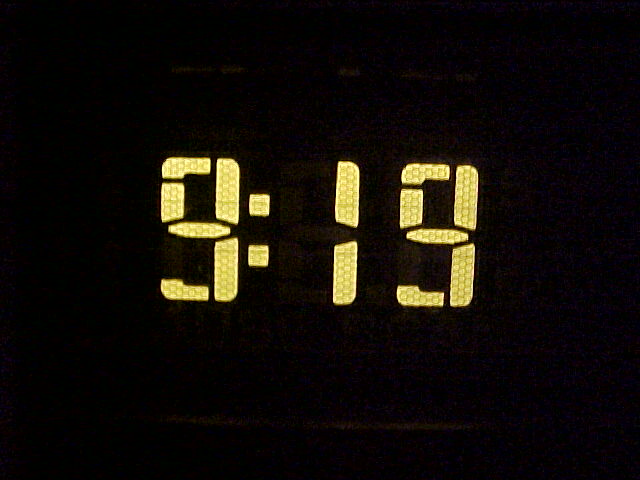The image depicts a close-up view of a digital alarm clock in a very dark setting. The background is a deep black, and against this, the bright yellow digital readout of the time "9:19" stands out prominently. The digital numbers consist of small dots arranged in lines, creating a textured appearance. The colon separating the hour and minute digits is spaced notably far from the "1". A faint rectangular shape, possibly the illuminated border of the clock face, can be seen reflecting the yellow light from the digital numerals, though details of this shape are barely visible due to the low lighting. The overall impression is that of a digital clock face glowing in a dark room, displaying the time as 9:19.